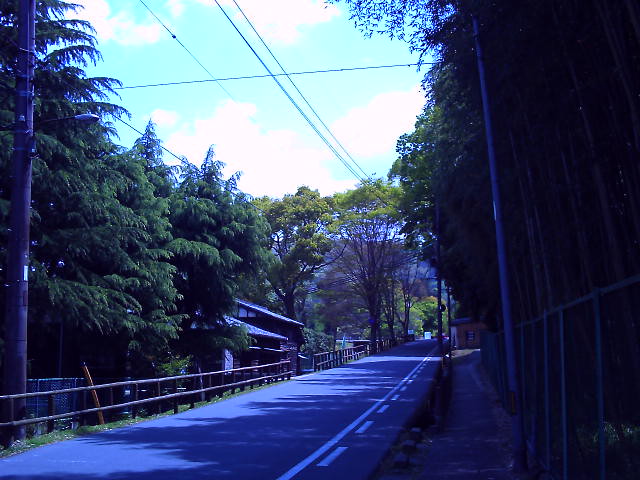This atmospheric photo captures a tranquil street scene either at dawn or dusk, characterized by the fading or emerging light. The road, possibly a one-way stretch, features a combination of dashed and solid white lines along its blacktop surface. Flanked by towering green trees with thick brown trunks, the street is bordered by a variety of fences—one side showcases a wooden fence while the other is secured with a metallic wired fence. Some viewers noted that this metallic fence appears silver and higher compared to others.

A mix of residential structures is visible in the distance: homes on the left side and sporadic houses stretching further down the road. Specific details point to the homes having brown exteriors with green rooftops and white trims. 

Electric poles bearing power lines run parallel to the road, contributing to the rustic feel of the area. Sidewalks on both sides of the street, featuring gray blocks or bricks, add to the structured appearance of the scene. The blue sky, dotted with white clouds, enhances the peaceful atmosphere. On the left side near the houses, an orange pool noodle covers the bottom part of a wire, adding a peculiar but noticeable detail to the otherwise serene environment. Overall, this image captures a quiet, rural neighborhood road surrounded by the lushness of nature.